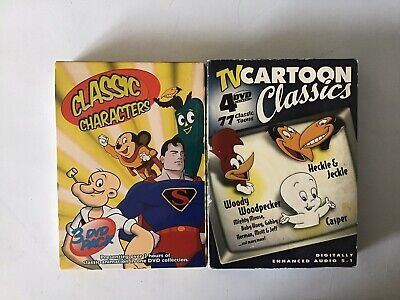This image is a landscape-oriented color photograph showcasing two vintage comic book-styled boxes featuring classic cartoon characters. The box on the left, with a golden cover, prominently displays a red oval-shaped text box reading "Classic Characters." It features iconic figures such as Superman in a dark blue tunic with a red 'S' emblem, Popeye the Sailor Man with his hands on his hips and a pipe in his mouth, Mickey Mouse in the center, and another forgotten green character. This box is vibrant and colorful, adding to its nostalgic appeal.

To the right, the black-and-white-themed box is titled "TV Cartoon Classics" and includes a white text reading "77 Classic Cartoons Set." The cover showcases Woody Woodpecker on the top left, the mischievous duo Heckle and Jekyll on the top right, and Casper the Friendly Ghost on the bottom, set against a cream and gray background. Both boxes collectively evoke a sense of nostalgia through their detailed representation of beloved, timeless cartoon characters.